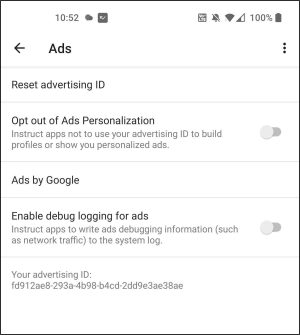The image depicts a smartphone screen displaying the "Ads" settings menu. The status bar at the top of the screen shows the following indicators: Cloud icon at 10:52, Wi-Fi and mobile signal icons with half signal strength, and a full battery icon.

The screen is divided into sections, each bordered by thin gray lines. There are five prominent gray lines: one below "Ads," another beneath "Reset advertising ID," the third under "Opt out of ads personalization," the fourth below "Ads by Google," and the last under "Enable debug logging for ads."

The main section contains several options and toggles:
- "Reset advertising ID" with a sub-option to reset your advertising ID.
- "Opt out of ads personalization," where the toggle switch is in the "Off" position, indicating apps are allowed to use your advertising ID to build profiles or show personalized ads.
- Below is the "Ads by Google" section.
- "Enable debug logging for ads," where the toggle switch is also "Off," meaning apps are not allowed to write ad debugging information, such as network traffic, to the system log.

At the bottom of the main section, your unique advertising ID is displayed: "FD912AE8-293A-4B98-B4CD-2DD9E3AE38A."

All text on the screen is black against a white background, providing clear contrast and readability.